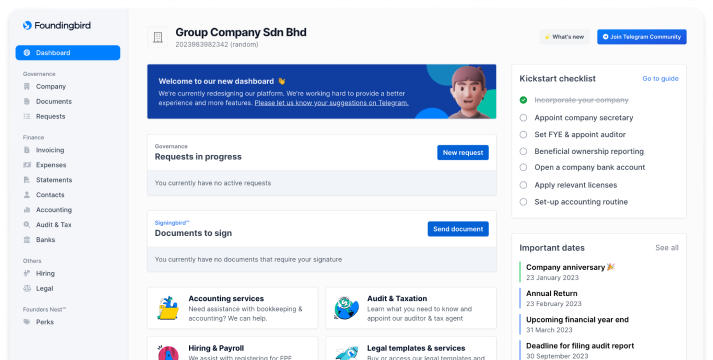A comprehensive and detailed caption of an image revolving around a business management platform might be:

---

"Introducing the new company dashboard, meticulously designed to streamline your corporate governance and administrative tasks. Welcome to a hub that combines the essential elements for managing your enterprise efficiently. Here, you can find:

- **Corporate Management:** Set up and maintain detailed information about your company, appoint a company secretary, and set financial year-end dates. Facilitate beneficial ownership reporting and other crucial administrative tasks.
- **Banking and Licenses:** Guidance for opening company bank accounts and obtaining relevant licenses, ensuring all your financial setups are compliant with regulations. 
- **Accounting:** Establish and follow through with an effective accounting routine, with available assistance for bookkeeping and accounting needs.
- **Governance:** Manage requests in progress, track new requests, and monitor important dates. There’s also functionality for appointing auditors and overseeing taxation requirements.
- **Document Management:** A section dedicated to signing documents electronically. Easily send documents and track those that require signatures.
- **Service Offerings:** Reporting services and robust document management to keep all your essential files organized.
- **Additional Features:** Functions for invoicing, tracking company statements, contracts, hiring, legal concerns, and other management tasks. Access to founder news and exclusive company perks.
  
The user-friendly interface ensures that all of your company's critical operations are just a few clicks away, making navigating complex processes easier than ever.”

---

This detailed caption encapsulates the breadth and utility of the business management platform as presented in the initial voice caption.